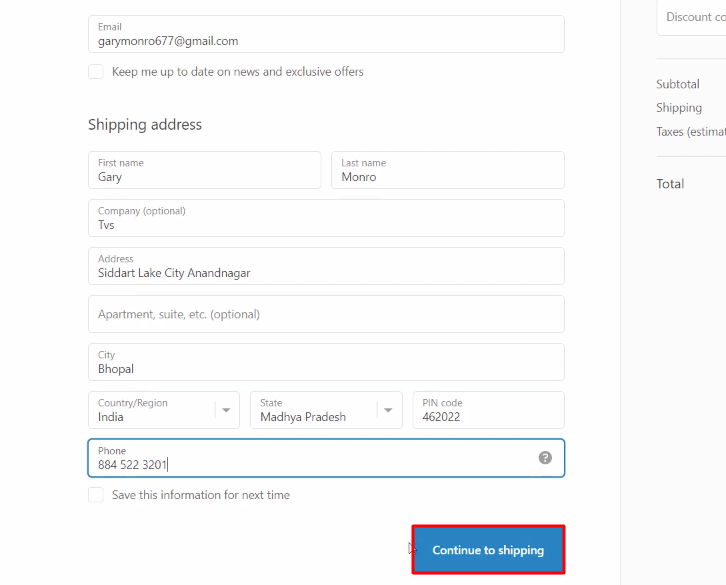This screenshot captures a segment of a website featuring a completed form. At the top of the form, there's an 'Email' field populated with "garymonroe677@gmail.com". Beneath that, a checkbox labeled "Keep me up to date on news and exclusive offers" is visible. Following is a section titled 'Shipping Address'.

The 'Shipping Address' section comprises several fields: the first row features 'First Name' and 'Last Name' fields filled with "Gary" and "Monroe", respectively. The subsequent 'Company (optional)' field contains the entry "TBS". The 'Address' field is filled with "Sedort, Lake City, NN Nagar". Below that, the 'Apartment, suite, etc.' field is left blank. The 'City' field contains "Bhopal". Further down, three side-by-side dropdown menus detail the country, region, and postal information: 'Country/Region' is set to "India", 'State' to "Madhya Pradesh", and 'PIN Code' to "462022". 

A 'Phone' field is also present but not filled in the screenshot. At the bottom of the segment, there's a blue "Continue to shipping" button encircled in red, likely indicating the next step in the form submission process.